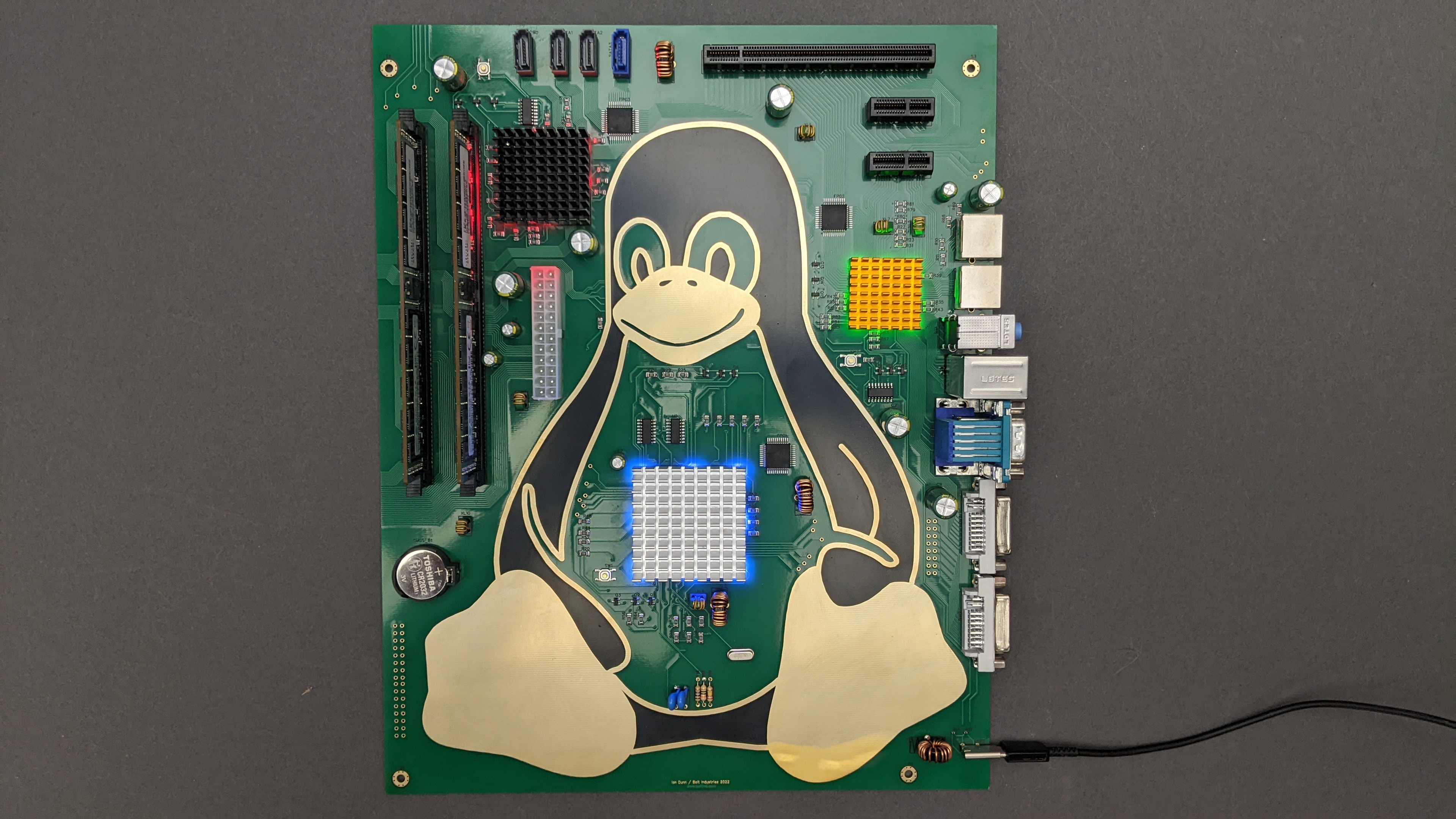In this intricate image, a green motherboard, likely part of a computer or laptop, serves as the backdrop. The motherboard bristles with various components such as transistors, hard drives, disks, and other internal parts essential to computer function. Superimposed on this green circuit board is a striking illustration of a penguin. This penguin has a black interior with a yellow outline, large upturned yellow feet, and a yellow beak. Its eyes are detailed with green irises, black pupils, and white borders. In the center of the penguin's belly is a lit-up square featuring a grid pattern with white and gray elements, bordered by blue lights. Additionally, there is a noticeable yellow square to the right of the penguin and a black square to the left of its head. The entire scene is set against a cohesive gray background, with a power cord located in the bottom right corner, hinting at the device's connectivity.